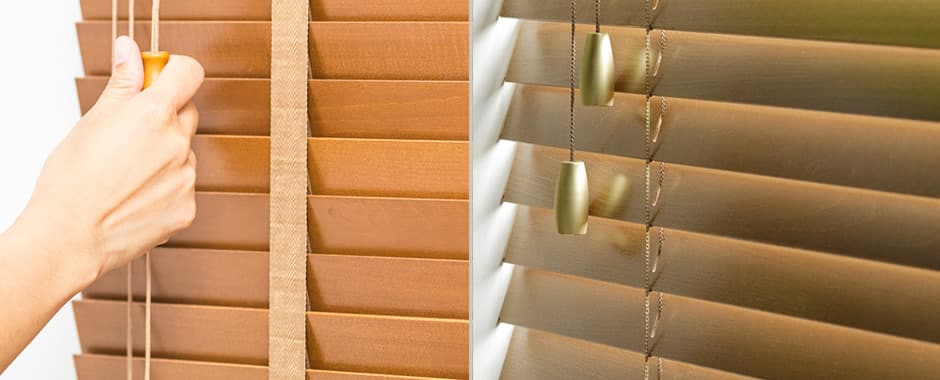This photograph showcases a comparative advertisement for wooden slatted window blinds, depicted through two separate images divided by a light grey line. The image on the left features a close-up view of a hand gripping the light tan pull cord to adjust the blinds, which are closed upward. The blinds here are made of a lighter reddish-brown wood, with a light tan ribbon running through the middle. The pull handles are light tan as well, blending seamlessly with the overall tone. Contrastingly, the right image displays a different variation of these blinds, characterized by darker wood and darker plastic or wood pole stops. These blinds, adjusted in a top-down orientation, allow sunlight to filter through the slots, with the string running through them being gold-colored. The pull handles on this side are iridescent gold, reflecting the sunlight. The illustration effectively contrasts the functionalities and aesthetics of the two blind sets under similar lighting conditions.